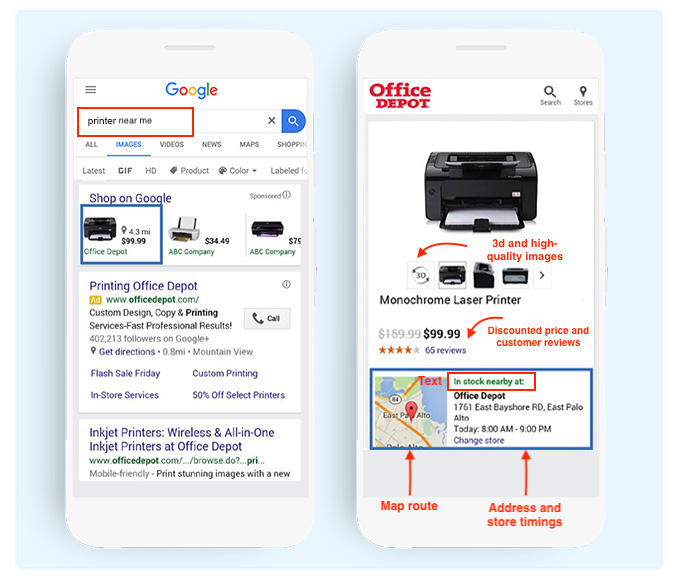A pair of detailed screenshots displayed side-by-side on a mobile device. The left screenshot shows a Google search result for "printer near me," with the Images tab selected. A red rectangle highlights a specific search result, emphasizing an Office Depot-sponsored link for a printer priced at $99.99 and located 4.3 miles away. Below this, two more printers are visible, along with an additional ad featuring Office Depot details and another printer result.

The right screenshot opens the highlighted Office Depot link, revealing a monochrome laser printer priced at $99.99. The page includes a product image and a map at the bottom, showing the store's location. Red text and arrows throughout the screenshot annotate and point out various elements and features of the webpage.